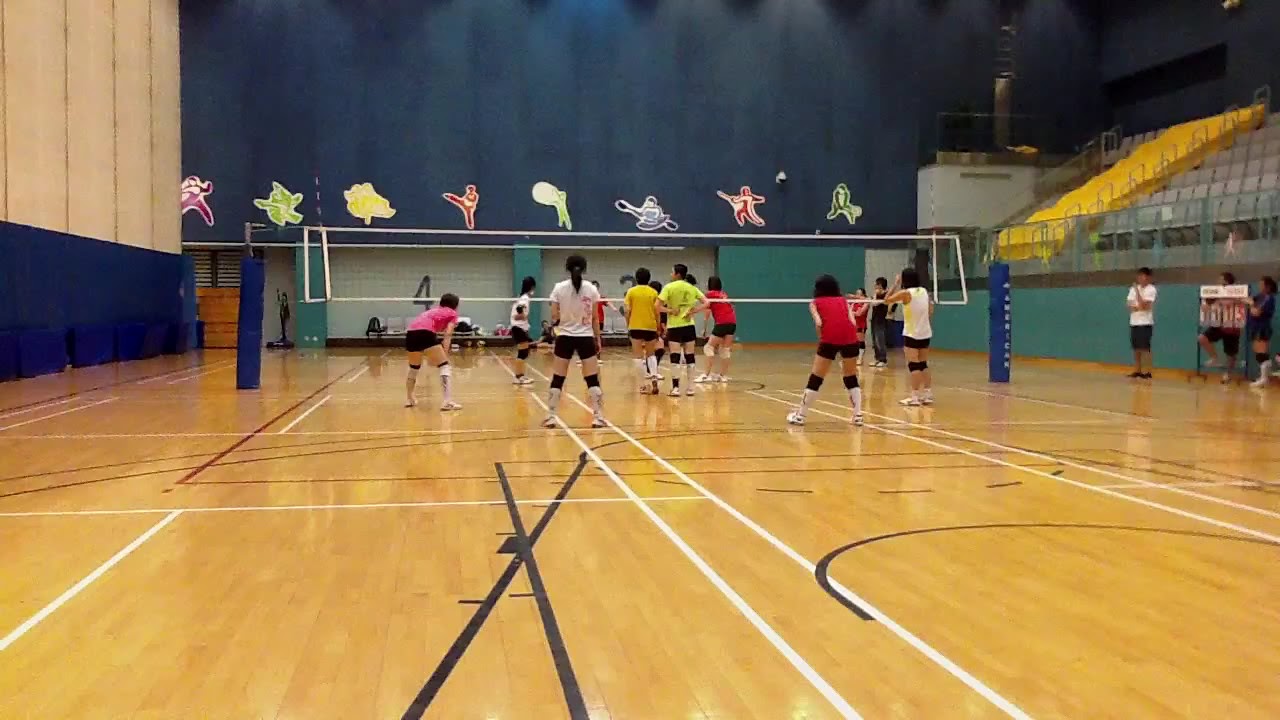In this indoor photograph, we see a volleyball practice or game setting, likely in a school gymnasium temporarily repurposed from a basketball court. The players, all girls with black hair, are positioned on either side of a central net, appearing to await the start of a match. Each player sports black shorts paired with various brightly colored shirts, including shades of white, red, pink, yellow, light green, and purple. Black knee pads accompany their attire. 

The camera captures the scene from behind a group of players in the foreground, giving a clear view of the net and the opposing team. To the right, a person, possibly a coach, wearing a white t-shirt and black pants, oversees the activity. The stands to the upper right remain empty, suggesting the game is either informal or a practice rather than a public event. 

The gymnasium features a light brown basketball court with distinct black and white line markings, and the background showcases a black wall adorned with various images of athletes engaged in sports such as tennis, baseball, kayaking, and karate. A partially visible, unreadable sign appears behind the white-shirted person. The overall composition centers around the net and the players, vividly capturing the preparatory calm before the action commences.